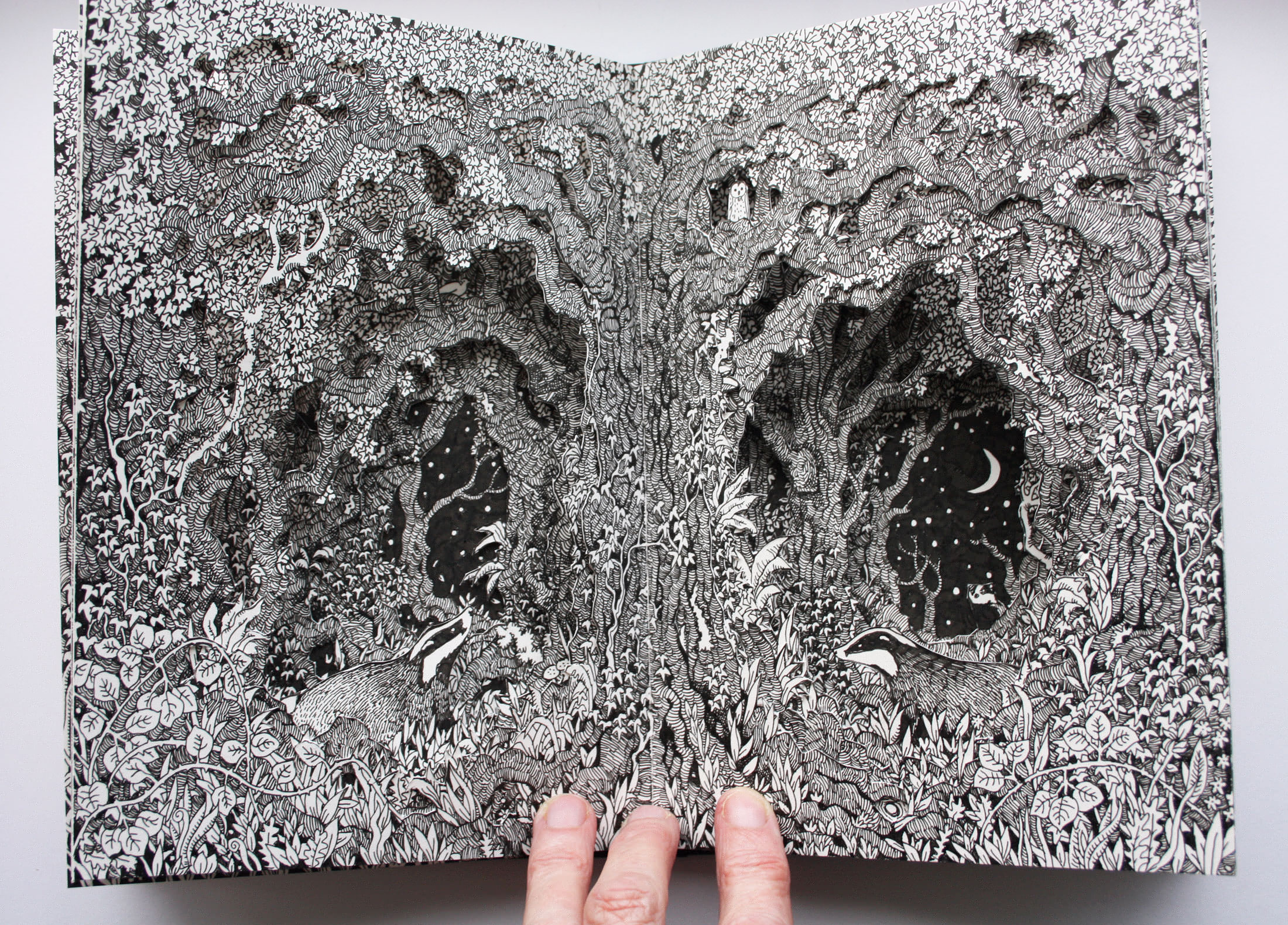This image is an intricately illustrated black and white drawing spanning two open pages of an art book. Three fingers at the bottom hold the book open, revealing the detailed artwork. The central focus is a tree that fans out into flowering foliage and branching vines at the top. At the bottom of the illustration, small bushes and grass surround two honey badgers positioned on either side of the tree. Above the badgers is a cut-out hole in the page, adding a three-dimensional effect and revealing a similarly drawn illustration on the subsequent page. This layering continues for at least three or four levels, each with its own intricate forest-like details, culminating in a final page depicting a starry black sky with a small crescent moon on the right side. The scene exudes a mesmerizing, almost fantastical quality, accentuated by the intricate detailing and the layering effects of the paper cut-outs.